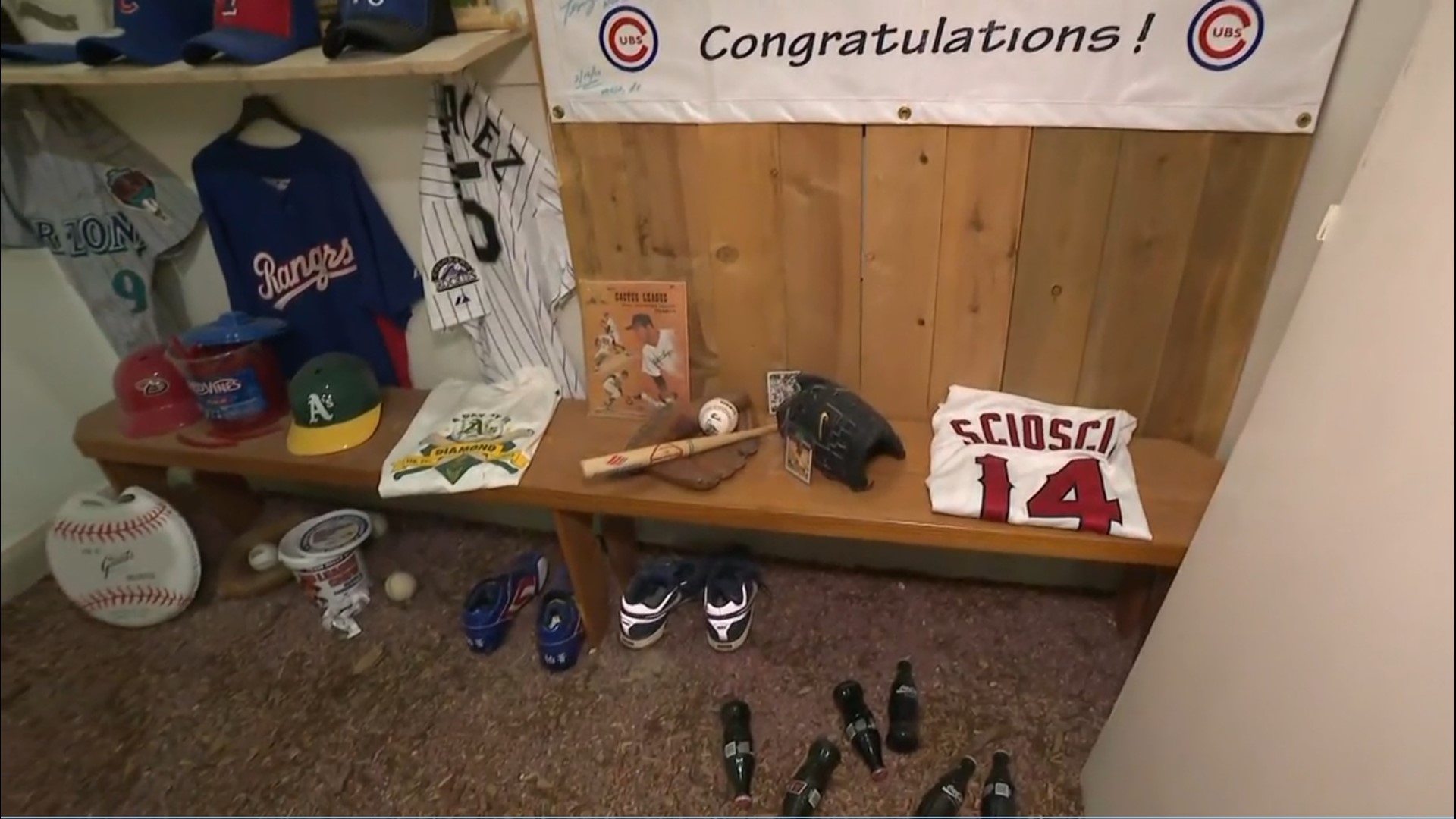The image depicts a detailed scene inside a locker room, resembling a professional baseball player's space filled with diverse memorabilia and gear. The floor is covered with a brownish-beige carpet, scattered with several baseballs, pairs of baseball shoes—including black and white as well as navy blue—and glass Coca-Cola bottles, some of which appear unopened. The walls are a mix of wooden panels and white paint, adorned with various baseball jerseys. Prominently, there's a white striped jersey with the number 5, a gray jersey marked with the number 9, a navy blue shirt that reads "Rangers," and another that appears to be a Colorado Rockies jersey with the name "Gonzalez." A banner above a wooden bench features the Chicago Cubs emblem in its iconic blue, red, and white colors and boldly congratulates someone. On the bench lies a white jersey with the possibly incomplete name "SCIO SCI" and the number 14 in red text, accompanied by a brown catcher's mitt, a black knee pad, a wooden bat, and a baseball. Behind the bench is a poster-sized baseball card, and nearby, a white bag shaped like a baseball and numerous knickknacks add to the clutter. The ledge above holds an assortment of four baseball caps, highlighting the array of baseball memorabilia that encapsulates the essence of the sport in this locker room.